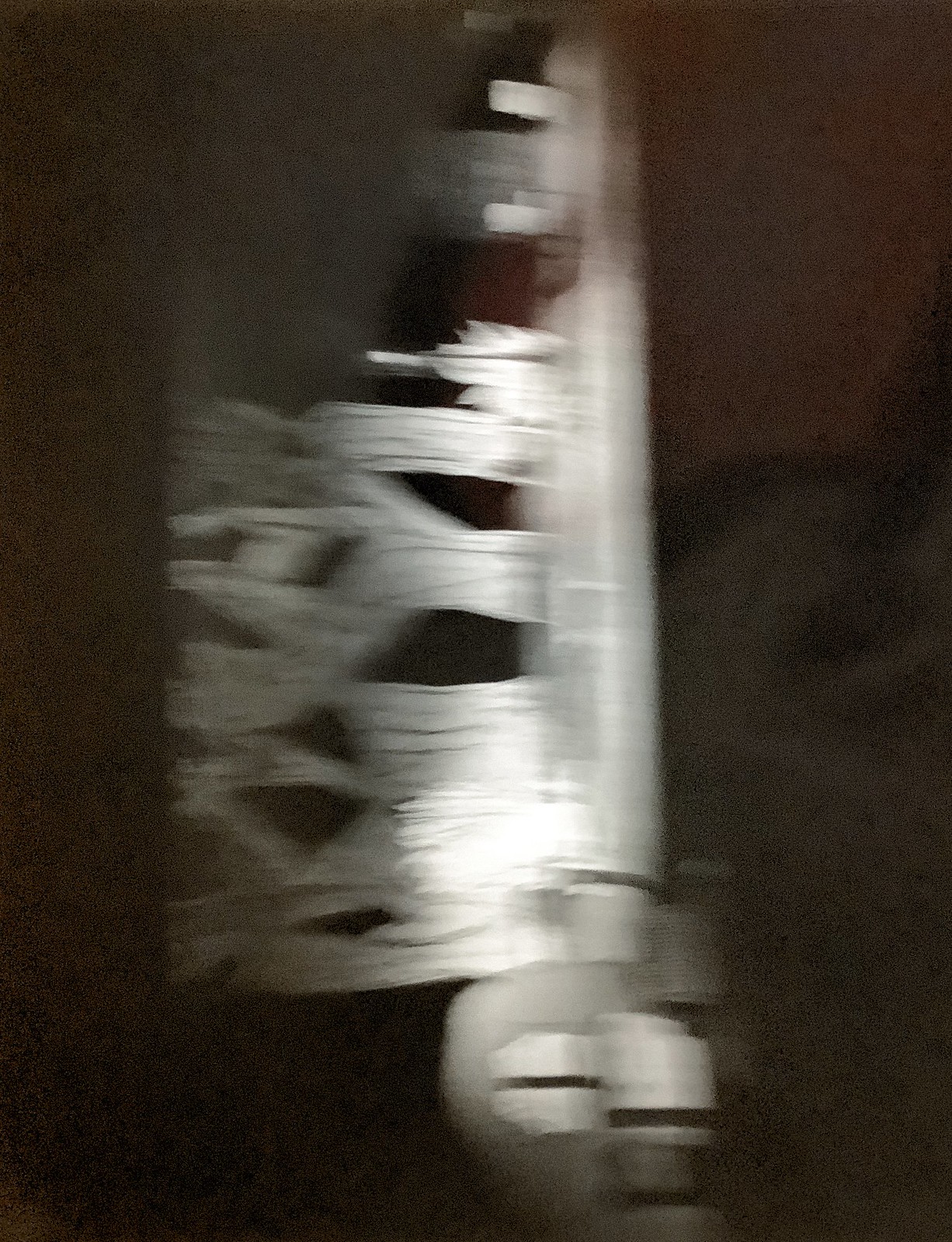Vertical, slightly blurry night vision image captures a monochromatic scene. A distinct U-shaped object rests at the bottom of the frame, cradling a cushion-like item marked by a prominent black line. A road illuminated by an unseen light source stretches upwards, flanked by trees and brush on the right-hand side. The foreground is enveloped in dense black, contrasting with a lighter gray, reflective night sky, typical of night vision visuals.